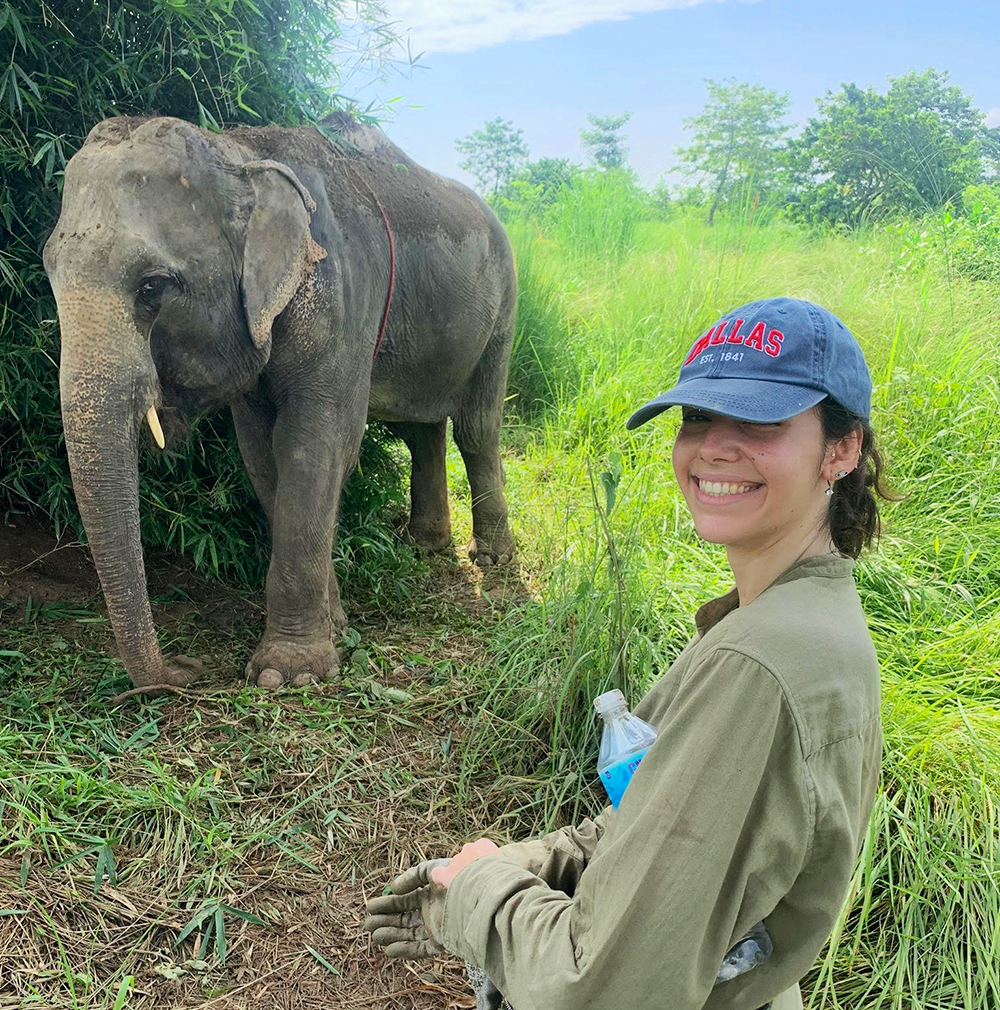The photograph features a detailed scene set in a grassy, jungle-like environment filled with tall greenery and numerous trees. Dominating the left side of the image is a baby elephant, distinguishable by its relatively small size and single tusk. The elephant has some dirt visible on its ear and trunk, and its trunk is resting on the ground. A tree and a mountain are faintly seen in the backdrop.

In the bottom-right corner of the squared photograph, a woman stands facing sideways but smiles directly at the camera. She is a white woman who appears to be in her twenties, donning a blue denim baseball cap embroidered with "Dallas" in red and "established 1841" in white. Multiple earrings adorn her ears, and she has dark brown hair. She wears a long-sleeve, button-up, safari-like shirt in a grayish-green hue, with a large brown glove on her right hand. Tucked in the crook of her left arm is a plastic single-use water bottle featuring a white cap and a blue label. The background consists of dense trees and tall grass reaching above the woman's head.